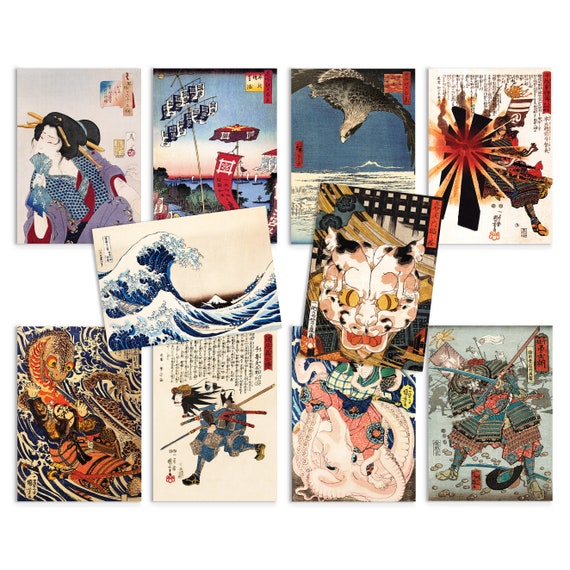The image is a rectangular collage comprised of ten smaller pictures, arranged in a structured format. There are four pictures aligned horizontally at the top, four pictures similarly arranged at the bottom, and two pictures placed at the center with a white gap separating them. Each segment is bordered by minor gaps.

The first image in the upper left corner features an Asian woman, possibly Japanese or Chinese, with her hair elegantly pinned up using sticks. She is dressed in a bluish garment and appears to be holding a fan near her face, partially obscuring her expression. 

Among the images in the middle section, the left one vividly captures a dynamic scene of the ocean, highlighting a large wave on the verge of crashing. The intricate details of the wave depict the moment's intensity and power.

The content of the remaining seven images is ambiguous, as they each illustrate distinct scenes or subjects that are not easily identifiable. The collage collectively presents a rich and varied visual narrative, blending diverse elements that invite closer inspection and interpretation.